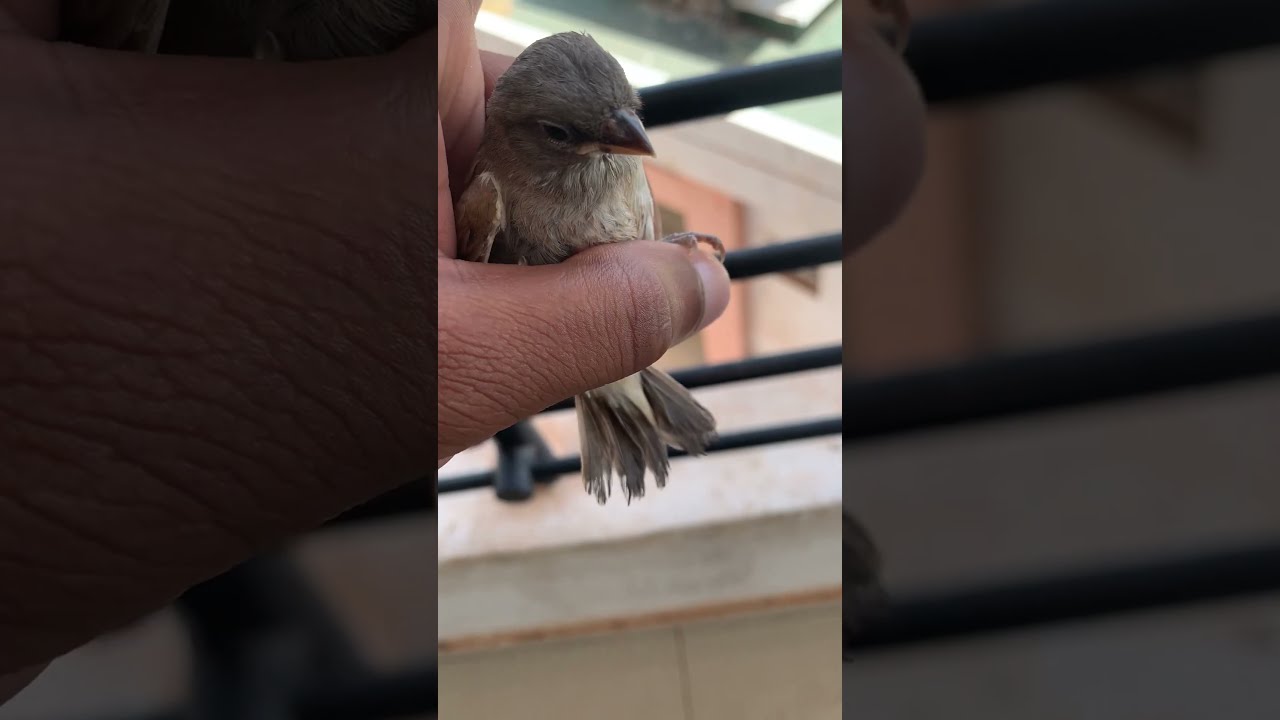The photograph is divided into three vertical sections, with the first and third sections being darkened and blurred close-ups of the central image. The central section shows a dark-skinned man's hand gently holding a tiny bird between his thumb and index finger. The bird, with a head of gray feathers, dark beak, and a breast and wings covered in light gray or white feathers, appears calm and relaxed, its head tilted slightly to the left. The background reveals a balcony area, with a black banister and a white-painted base, and beyond that, blurred buildings and possibly a rooftop scene. The overall atmosphere suggests tranquility, with the bird seeming content and unafraid in the man's grasp.